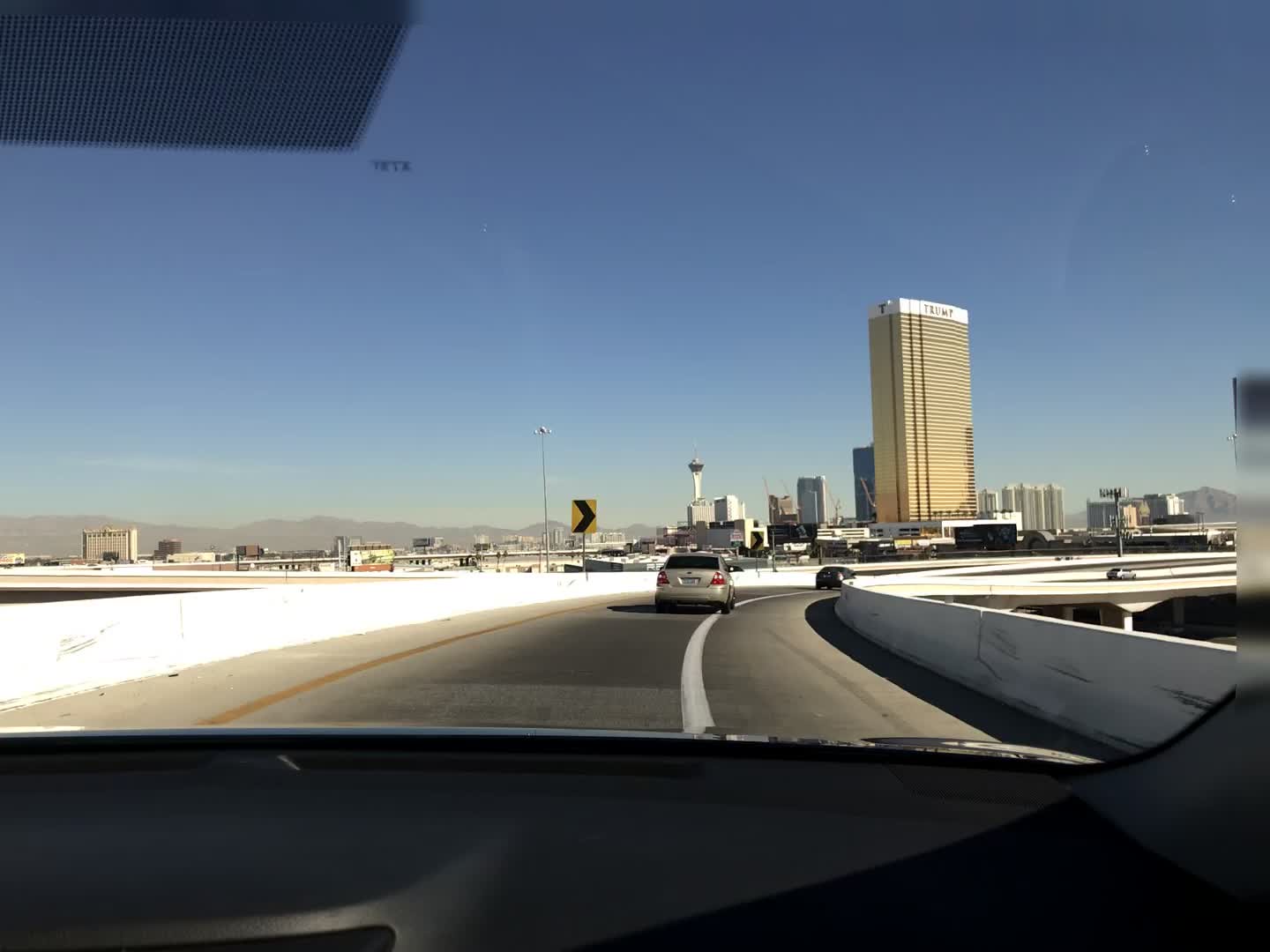The photograph, captured in a landscape orientation through the windshield of a car, presents a scene from the highway in a bustling city. The upper left-hand corner shows part of a black visor, while the bottom edge reveals a black dashboard. The sky above is blue and clear, though tinged with light smog. Ahead, the highway, currently a one-lane ramp, is delineated by a white jersey barrier on the right and a yellow line on the left. A conspicuous sign indicates an upcoming curve to the right. Two cars, including a tan one and a gray SUV, are visible ahead of the vehicle taking the picture, along with another car further in the distance. Prominently, a space needle-like building with a tall thin structure and a round top floor rises beyond the highway, alongside a notably tall rectangular gold building with a white top, which stands about five times taller than the surrounding gray and black buildings. In the far distance, faint outlines of mountains add to the urban landscape.